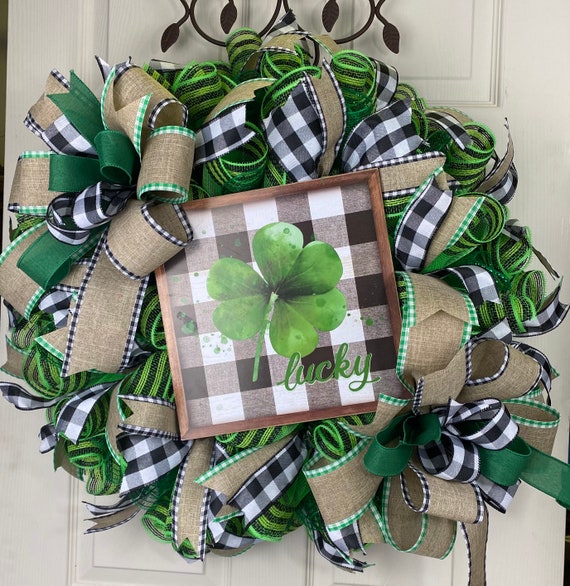In the image, an off-white door with four visible panels serves as the backdrop for a festive St. Patrick's Day wreath. At the top of the door, a black metallic leaf structure holds the wreath in place, though only part of it is visible. The wreath itself is a handmade, circular arrangement of various ribbons. Dominating the left side is a large bow comprised of striped light kelly green ribbon, a burlap ribbon with a black and white plaid edge, and a darker green ribbon. The wreath is adorned with additional green spiraled ribbons, black and white buffalo plaid ribbons, and brown ribbons with plaid accents.

In the center of the wreath is a brown wooden picture frame with a background featuring a black, white, and gray checkerboard pattern. At the heart of this frame is a watercolor-style depiction of a green three-leaf clover. Below the clover, in green text with a fancy font, is the word "Lucky." The cohesive design and detailed elements of the wreath, such as the meticulously hemmed ribbons and the vibrant green bows interspersed throughout, contribute to its charming homemade appearance ideal for St. Patrick's Day celebrations.